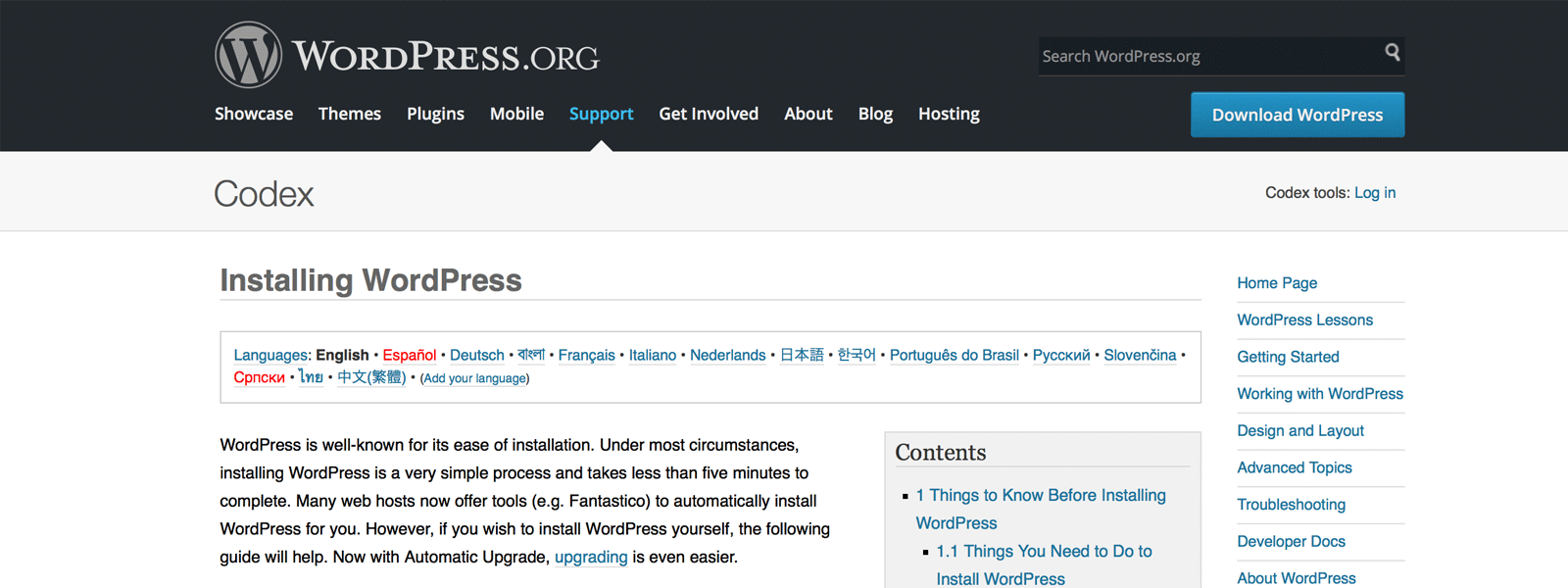This is a detailed description of a specific page on the WordPress.org website, guiding users on how to install WordPress. 

At the top of the page, there is a black navigation bar. On the top left, the WordPress logo appears as a white "W" inside a circle, next to the "WordPress.org" text. Below this, there is a series of navigational tabs in a white font, reading from left to right: "Showcase," "Themes," "Plugins," "Mobile," "Support" (highlighted in blue to indicate the current selection), "Get Involved," "About," "Blog," and "Hosting." On the right end of the black bar, a blue pill-shaped button is labeled "Download WordPress."

The main content on the page begins with a category label "Codex" on the left, and options "Codex Tools" and "Log In" in blue text on the right. Below that, a heading reads "Installing WordPress," followed by instructions about selecting your language. English is selected by default, but other available languages, including Español, Deutsch, and Français, are displayed with links in red and blue text.

The instructional text starts with a comforting description of the installation process: "WordPress is well-known for its ease of installation. Under most circumstances, installing WordPress is a very simple process and takes less than five minutes to complete. Many web hosts now offer tools, e.g., Fantastico, to automatically install WordPress for you. However, if you wish to install WordPress yourself, the following guide will help you."

To the right, there is a blue box titled "Contents" at the top, listing essential topics underneath. These topics are: "One Thing to Know Before Installing WordPress," followed by a subcategory, "Things You Need to Do to Install WordPress."

On the far right, there is a vertical, blue-font list of selectable categories: "Homepage," "WordPress Lessons," "Getting Started," "Working with WordPress," "Design and Layout," "Advanced Topics," "Troubleshooting," "Developer Docs," and "About WordPress."

This comprehensive layout aims to guide users seamlessly through the process of installing WordPress, covering all necessary steps and resources.